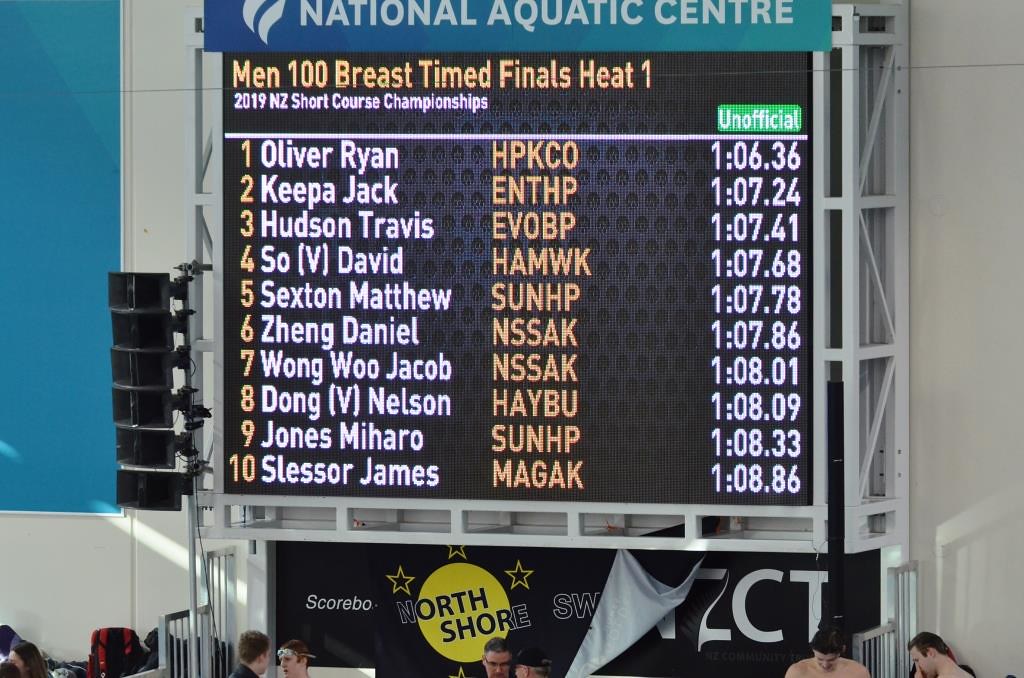The image captures a detailed photo of an LED scoreboard situated in a gymnasium-like environment, likely housing a pool given the context. The top section of the scoreboard prominently displays "National Aquatic Centre" in white uppercase letters against a blue-teal background. Below it, the illuminated scoreboard reads "Men 100 Breast Time Finals Heat 1" in yellow text, indicating the event being tracked. This is followed by "2019 NZ Short Course Championships" and the word "Unofficial" in a green and white font placed on the far right. 

The scoreboard lists competitors numbered from 1 to 10, starting with Oliver Ryan, with the names in white and the numbers in yellow. Each swimmer's time, mostly starting with the numeral 1, is also displayed in white, with the top time listed as 1:06.36. In the middle section, the teams or affiliations of the swimmers are listed in yellow. Below the scoreboard, the tops of athletes' heads and a white and blue section of the wall are visible, suggesting they are waiting for their turns or results. Loudspeakers are also seen attached to the poles supporting the scoreboard, indicating the setup is for announcing event details.